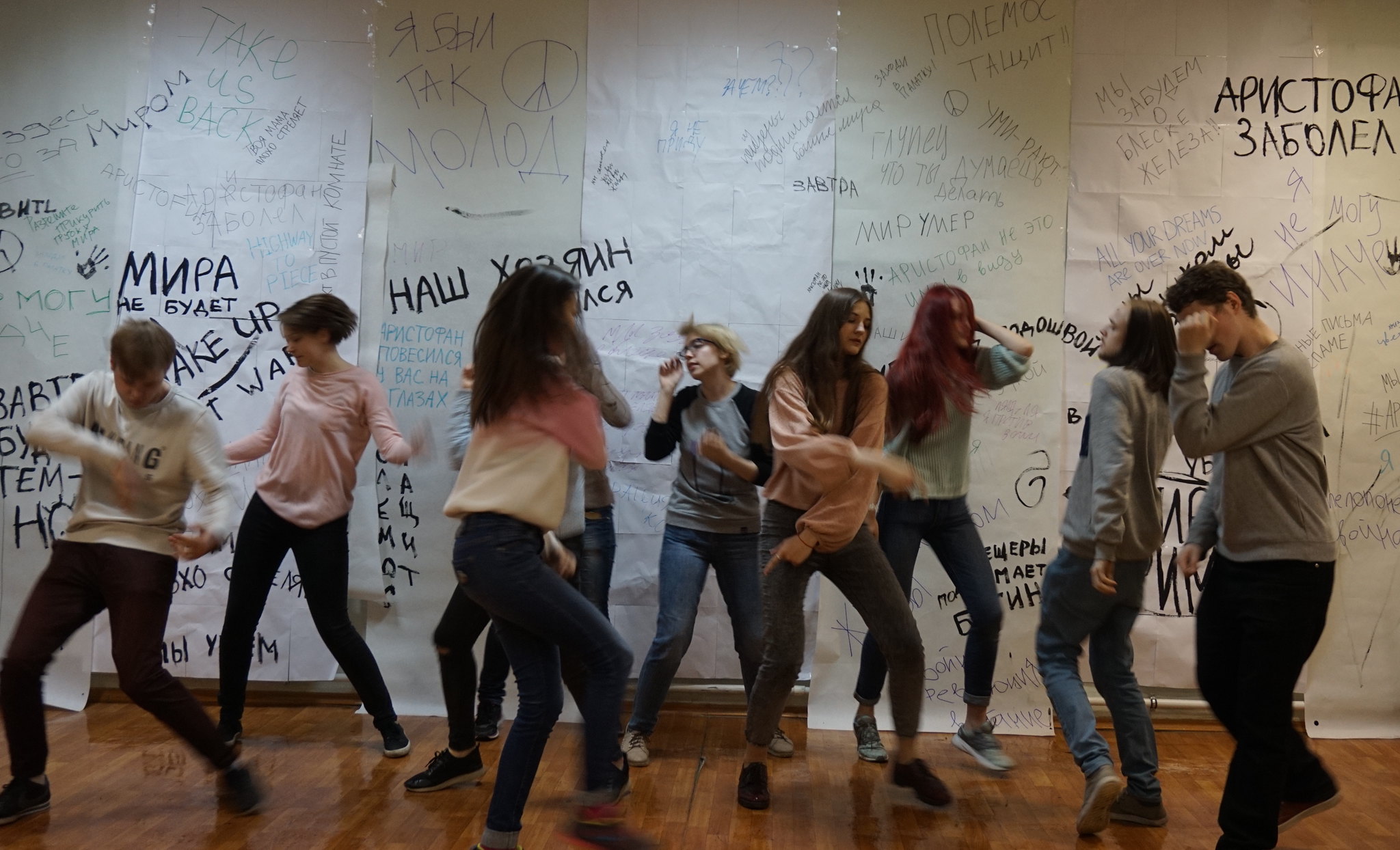The photograph captures a dynamic scene of 10 to 12 young people, likely teenagers or young adults around 18 to 19 years old, energetically dancing in a room with warm brown hardwood floors. They are dressed predominantly in dark pants or blue jeans, along with long-sleeve shirts and sweatshirts, and most are wearing sneakers. The background features large pieces of paper taped to the wall, covered with a mixture of handwritten text and symbols, predominantly in Cyrillic script, suggesting a Russian-speaking environment. Among the mostly black and blue ink writings, the phrase "take us back" stands out in English, written in green marker. One dancer, notably in the center of the image, is wearing glasses. The overall atmosphere is lively and spontaneous, reminiscent of an art gallery or a creative space.